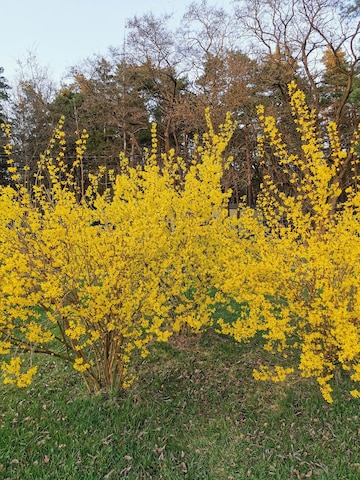This photograph captures a vibrant early spring scene, likely in a region with pronounced seasonal changes, such as the mid-Atlantic. In the foreground, two large forsythia bushes, around four to six feet tall, stand prominently. These bushes are adorned with bright yellow flowers on stringy stems that reach upwards, set against a green grassy field speckled with remnants of brown leaves. Behind the bushes, a variety of trees create a layered backdrop: a bare tree on the far right, a tree with lingering brown leaves, another with early yellow foliage, and a tree on the far left still holding onto its green leaves. The scene is bathed in natural light with a clear, cloudless blue sky overhead, signaling a crisp and pleasant day. The overall composition hints at the transition from winter to spring.